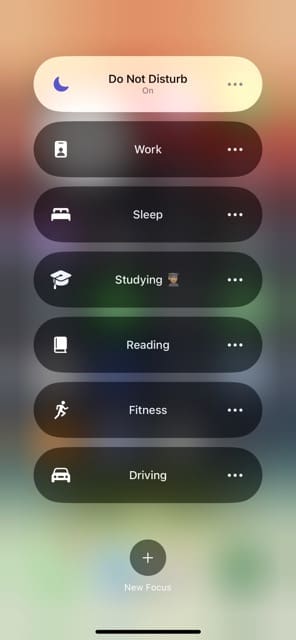The image appears to be a screenshot of the "Focus" settings on an Apple iPhone. At first glance, it consists of a list of seven different Focus modes, each within a horizontally elongated oval. These ovals are vertically arranged from top to bottom, with specific symbols and text indicating each mode.

1. The first oval, more opaque and white than the others, suggests it is currently active. It features a moon symbol on the left and three dots on the right. The text within this oval reads "Do Not Disturb is On."
2. The second oval, labeled "Work," displays a phone with a profile symbol on its left side.
3. The third oval, labeled "Sleep," includes a bed icon on the left side.
4. The fourth oval, "Studying," located around the middle of the screen, shows a graduation cap icon on the left.
5. The fifth oval, "Reading," has a book icon on its left.
6. The sixth oval, "Fitness," features a running man icon on its left.
7. The seventh oval, "Driving," shows a car icon on the left side.

All ovals besides the first one appear less highlighted, indicating they are currently off. At the bottom of the screen, there is a circular plus sign symbol followed by the text "New Focus," suggesting an option to create additional Focus modes. Each mode helps users concentrate on specific activities by curating notifications and other distractions accordingly.